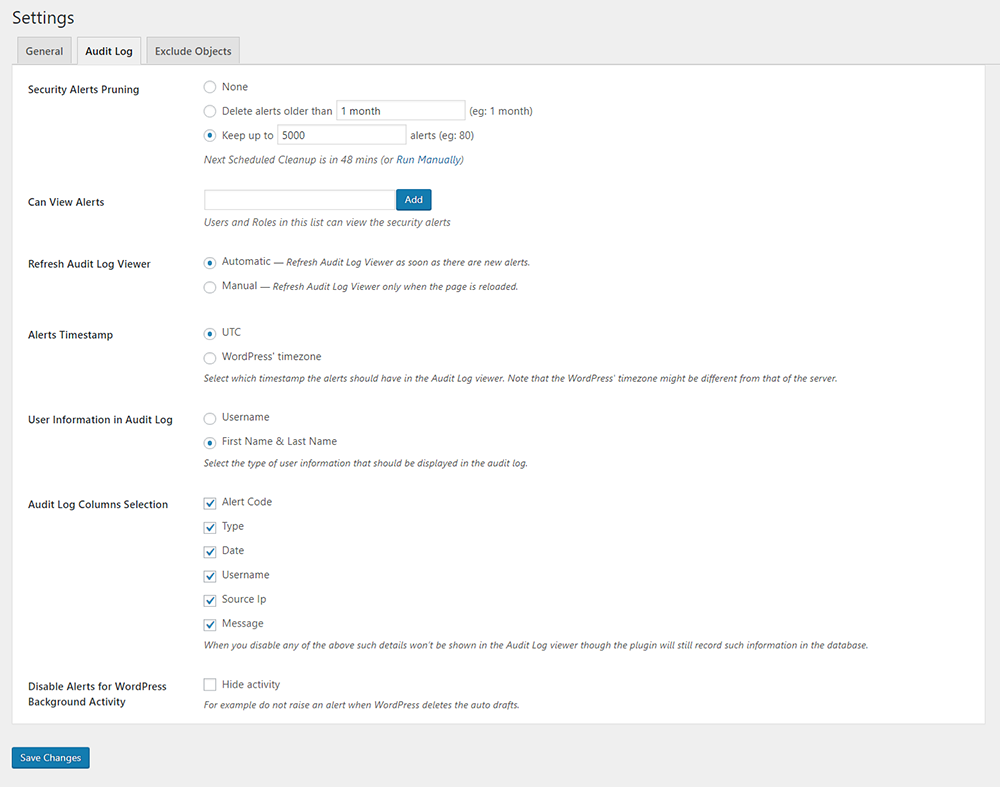This image depicts a detailed interface for managing security alerts within a system's audit log. Key sections include "Settings," "General," and "Audit Log," with a specific focus on "Security Alerts." The interface displays a configuration where security alerts for Texas are currently non-existent. It outlines the process of checking and deleting alerts older than one month, with a threshold to keep up to 5,000 alerts.

A blue square highlights the area where all users can view the security alerts. The checker prompts users to refresh the audit log viewer, now set to manual mode. There are options to select the timestamp format for alerts, either in UTC or according to the WordPress timezone, noting that the WordPress timezone may differ from the server's timezone.

User information in the audit log is configured to display the first and last names instead of usernames. The audit log columns are customizable, with options to include alert code, type, date, username, source of the page, and message. Disabling any of these will prevent the details from appearing in the audit log viewer, though they will still be recorded in the database.

An important note is to disable WordPress from showing back-end activity, such as auto drafts, and to save changes at the bottom of the interface.